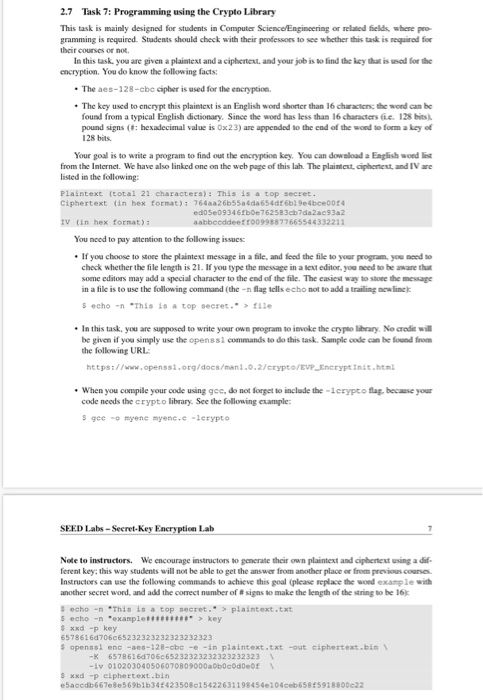**Task 2.7: Programming Using the Crypto Library**

This image depicts a structured document outlining tasks to be completed, focusing on programming with the Crypto library. At the top, the header "Task 2.7: Programming Using the Crypto Library" is displayed in bold black writing. Following this, the document explains in plain, non-bolded text the task's objective, detailing what the task is designed for, what actions the user will undertake, and the ultimate goal.

Midway down the first page, there is a gray box containing an example code snippet, rendered in a typewriter-style font. This box serves to illustrate the task requirements. The document continues with regular text after this boxed example, providing crucial points to focus on. This is followed by a bullet point that offers additional information.

Towards the end of the page, another example is given in code font but without the gray background. Another bullet point then instructs the user on specific steps for the task. To conclude the first section, a website link is provided, followed by a third bullet point explaining what to do when compiling the code.

At the top of the second page, a bold and underlined heading states "Seed Labs - Secret Key Encryption Lab." On the right side of the page is the number "7," indicating the page number. Beneath this, in bold, there is a note directed at instructors, followed by a brief paragraph in regular font suggesting instructional tips.

This paragraph is succeeded by a larger gray rectangular box, approximately twice the size of the first one, containing additional lines of code in the same typewriter-style font.